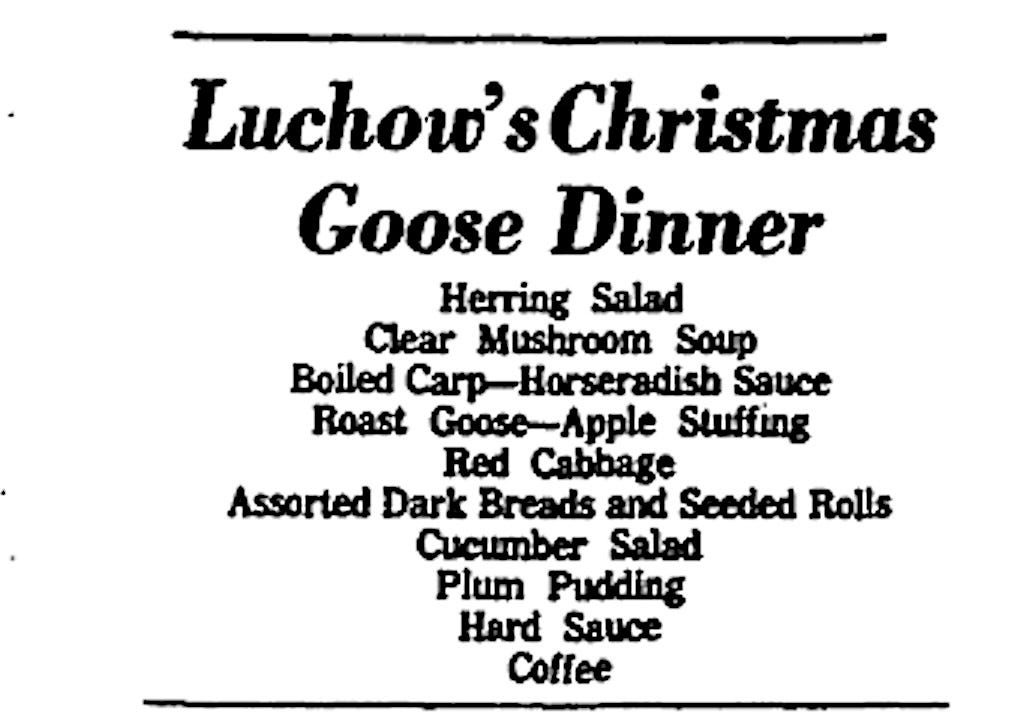The pixelated black and white image features a centered, text-only menu with a vintage appearance, possibly reproduced from an earlier era or cut from a magazine or newspaper. The title, in bold and larger font, reads "Lu Chow's Christmas Goose Dinner." Framed by horizontal black lines at the top and bottom, the menu items are neatly listed in a smaller, Times New Roman-like font, despite some blurriness due to the image being blown up. The menu includes: Herring Salad, Clear Mushroom Soup, Boiled Carp with Horseradish Sauce, Roast Goose with Apple Stuffing, Red Cabbage, Assorted Dark Breads and Seeded Rolls, Cucumber Salad, Plum Pudding, Hard Sauce, and Coffee.